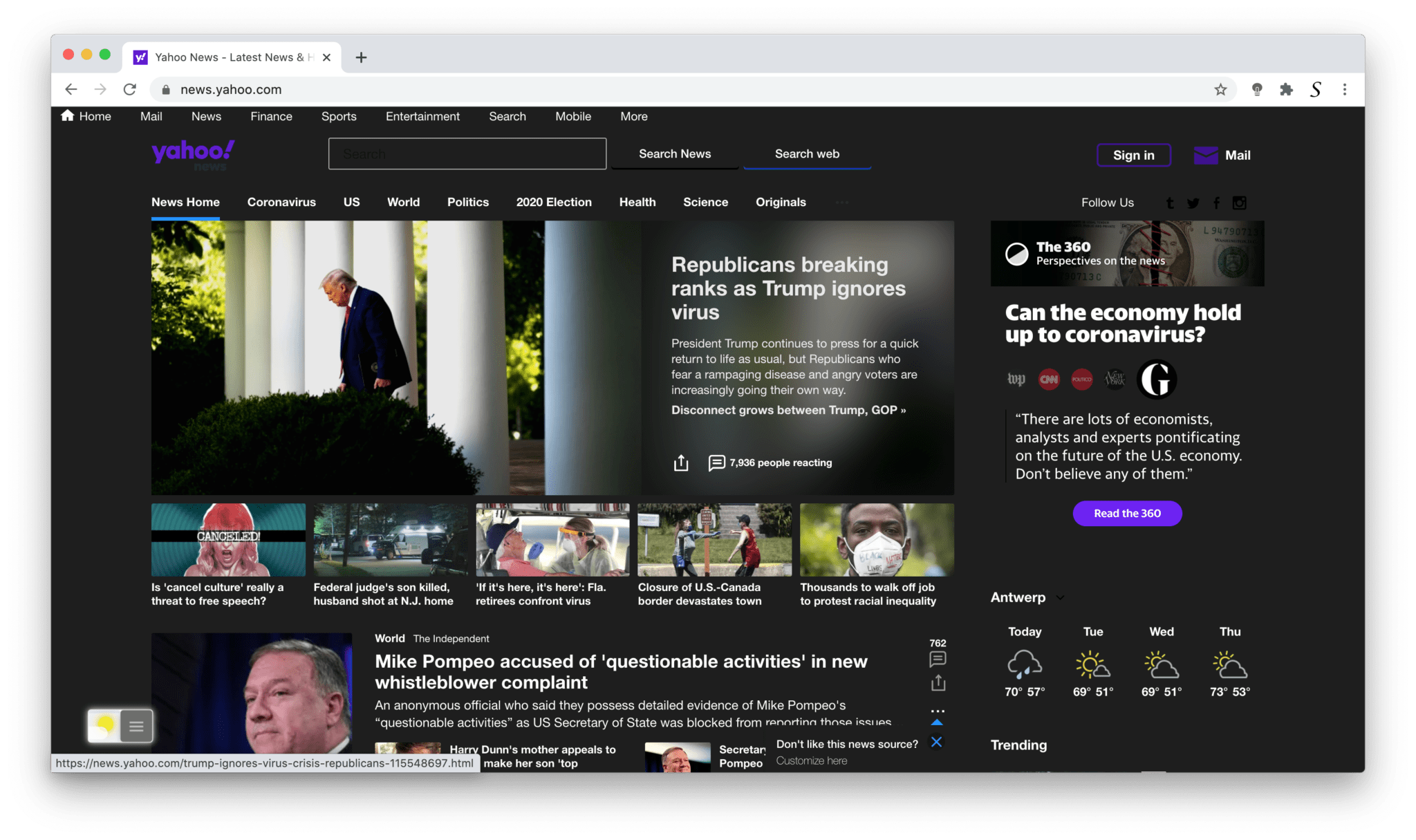The image displays a webpage from Yahoo News, characterized by its black background. At the top of the page are navigational options including Home, Mail, News, Finance, Sports, Entertainment, Search, Mobile, and More. Just beneath these options, there is a prominent search bar.

The main section of the page features a headline article accompanied by an image of Donald Trump. The headline reads: "Republicans Breaking Ranks As Trump Ignores Virus." The article preview notes that President Trump is advocating for a swift return to normalcy despite Republican concerns about a rampant disease and the potential backlash from voters. This divergence is described as a growing disconnect between Trump and the GOP.

Below the headline article, there are several other news stories, each paired with an image. These articles include:
1. "Is Cancel Culture Really a Threat to Free Speech?"
2. "Federal Judge's Son Killed, Husband Shot at New Jersey Home."
3. "If It's Here, It's Here: Florida Retirees Confront Virus."
4. "Closure of US-Canada Border Devastates Town."
5. "Thousands to Walk Off Job to Protest Racial Inequality."

The visual layout effectively highlights both the main story and additional articles that cover a wide range of pressing issues.